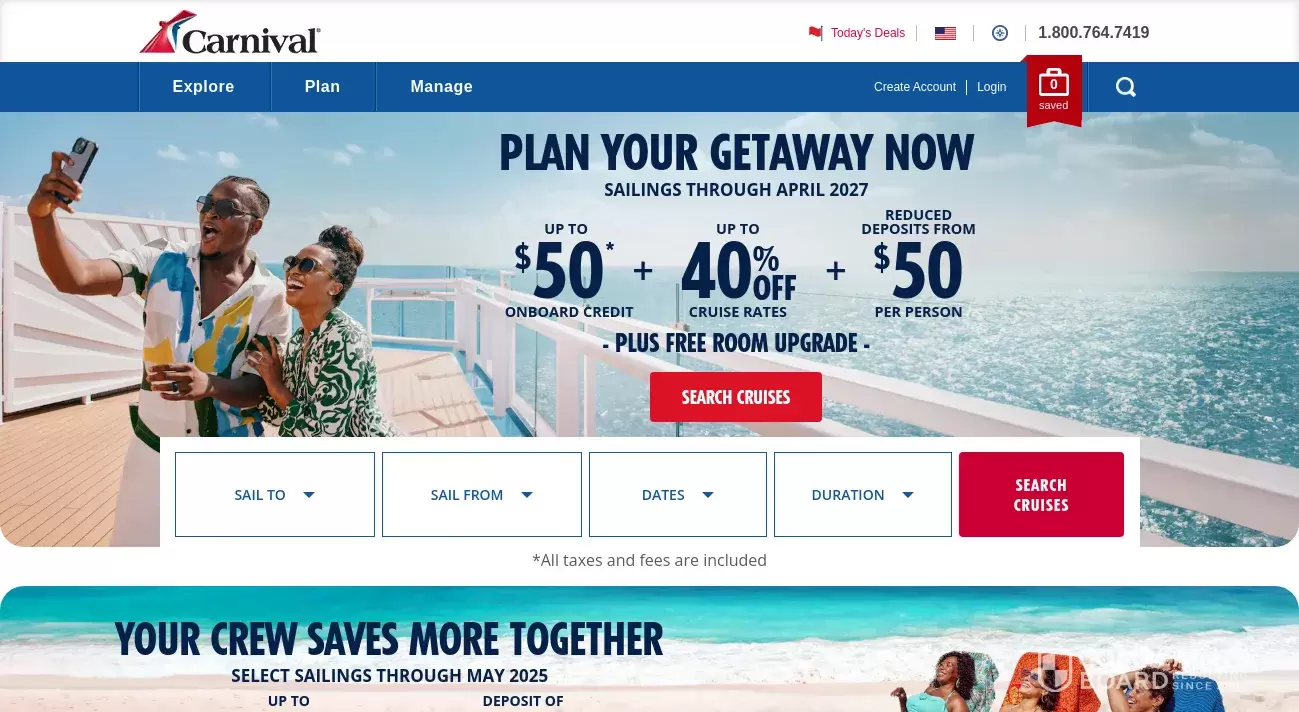Carnival Cruise Line Webpage Description:

The webpage of Carnival Cruise Line features a comprehensive and visually appealing layout designed for ease of navigation and customer interaction. 

**Top Navigation Bar:**
- **Logo:** On the left-hand side, there is the Carnival Cruise Line logo, depicting the bow of a ship in red, white, and blue.
- **Tabs on the Right-Hand Side:**
  - A red flag icon alongside the red text "Today’s Deals."
  - Blue text that reads "Sign Up and Save."
  - An American flag icon and a blue circle with a crosshair.
  - Contact number "1-800-764-7419" in black.

**Dark Blue Bezel (Navigation Menu):**
- **Left Side:** Clickable buttons in bold white text:
  - "Explore"
  - "Plan"
  - "Manage"
- **Right Side:** Clickable buttons in regular white text:
  - "Create Account"
  - "Log In"
  - A suitcase icon with a zero inside it; below it, the word "Saved" and a magnifying glass icon.

**Promotional Section:**
- **Carnival Cruise Line Credit Card:**
  - Features an image of a cruise ship with text: "Earn 20,000 Fun Points" in blue.
  - A red clickable button with bold white text says "Apply Now."
  - Disclaimer: "Terms Apply" in blue.

- **Limited Time Offer:**
  - A thick red rectangle displaying a countdown:
    - “Only” in white text, bold numbers for hours, minutes, and seconds, with labels HRS, MIN, and SEC respectively, followed by "Left."

**Main Content:**
- **Imagery:** Displays a family enjoying water activities near a building, people riding horses, and individuals leaning against a pier.

***Filtering Options:**
  - In a white bezel at the bottom:
    - "Sail To" with a blue border and a drop-down arrow.
    - "Sail From" with a blue border.
    - "Dates," "Duration," and a "Search Cruises" button in red with white text.

**Promotional Banner (Cyan Blue Background):**
- **Text with Thin Red Border:**
  - "No One Does" in blue.
  - "Limited Time Savings You’ll Love" in blue.
  - A red tag with the text "Sail" in white.

**Discount Offer:**
- "Cruises From" in blue with a strikethrough price of “579” and a discounted price of “289” in red.
  - An asterisk notation: "Per Person."
  - A red rectangle with white text that says "Search Cruises."

**Footer:**
- **Bottom Right Corner:**
  - "Complaints Board" in white text.
  - "Resolution Res Aliving Since 2004."

This detailed description of the Carnival Cruise Line webpage highlights its user-friendly features, promotional offers, and clear navigation, aimed at creating a streamlined user experience for customers.